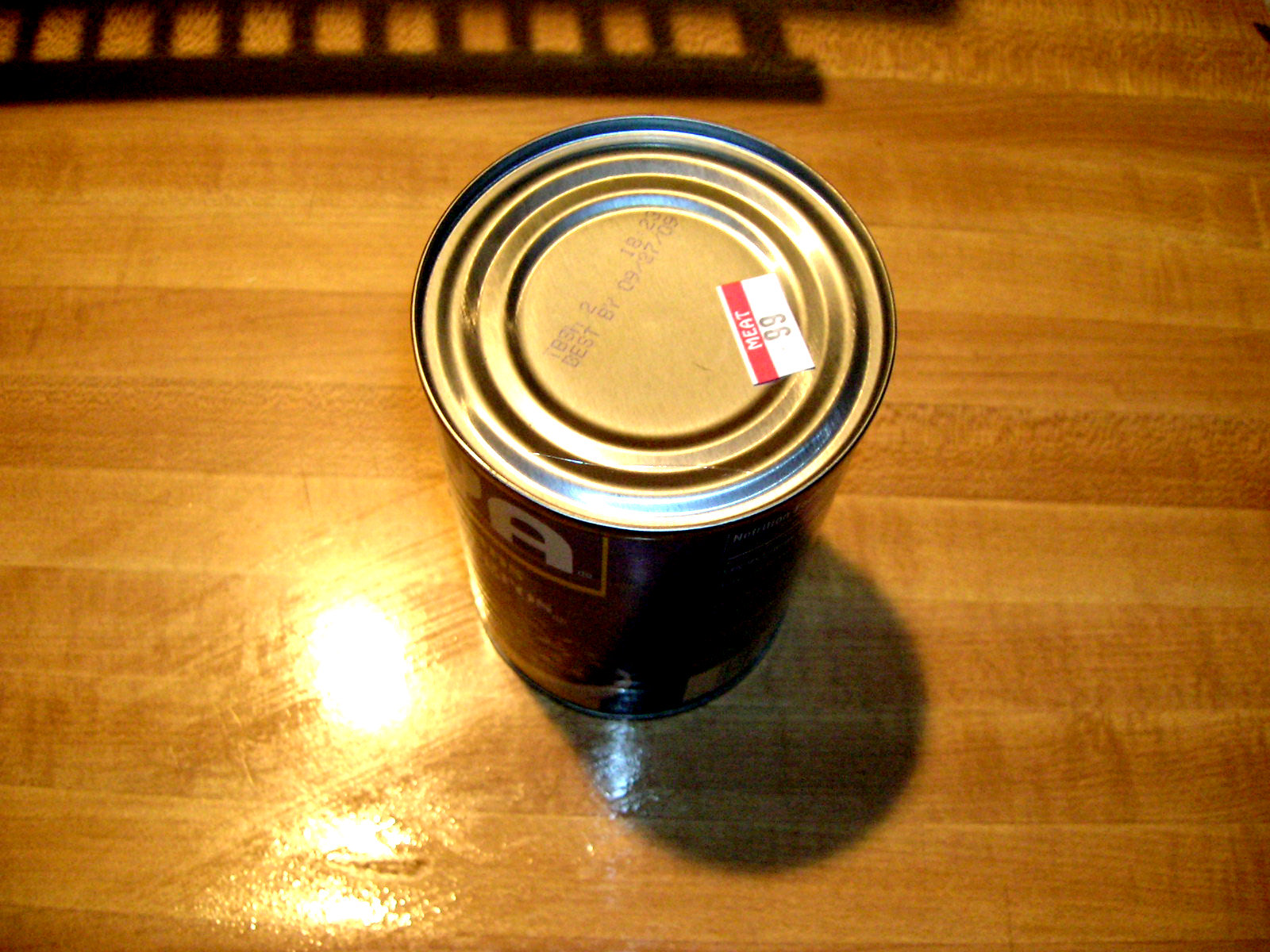This image, taken from an overhead perspective, features a tin can positioned centrally on a light brown, reflective, wooden surface, which is horizontally lined. The can, likely blue or dark in color, displays white letters "Y" and "A" encased in a yellow square on its front. The top of the can is silver and bears a sticker with "Meat" written in white against a red background, alongside the number "99." Additionally, the can's top is stamped with "Best By 090709." In the upper left portion of the image, a distinct shadow resembling a ladder or fence extends towards the center, contributing to the reflective interplay on the laminated wood. The scene also features a bright light source to the left of the can, enhancing the reflective quality of the surface and casting a prominent shadow of the can below it.